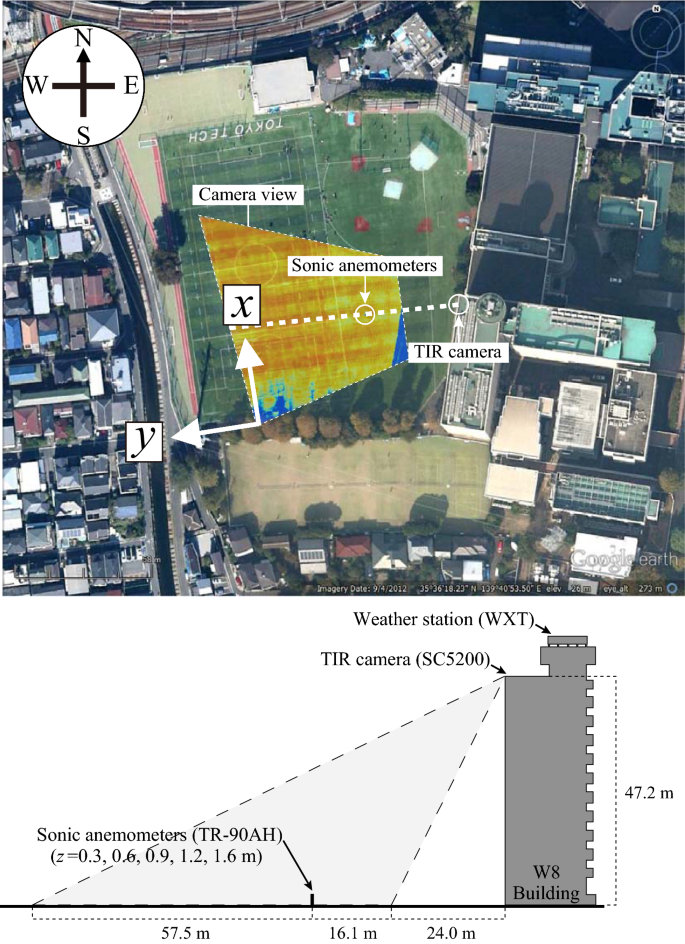The image is a detailed satellite view looking down onto a sports field, most likely a baseball diamond, which is clearly marked with white lines and the words "Tokyo Tech" in large white letters near the top left. The field is green with various angles and obscure shapes in orange and yellow drawn over it. Labeled components include "camera view," "sonic anemometers," "TIR camera," and "weather station," with respective arrows pointing towards these aspects. The X and Y axes converge at a 90-degree angle, marked towards the bottom of the image. Surrounding the field, on the right side, are large buildings with gray and light blue tops, while on the left side there are smaller buildings, appearing more like small houses. At the bottom of the image, there's a gray and white diagram depicting a building labeled "WV-8," described as being 47.2 millimeters high. This area is noted to be an outdoor, daytime shot and includes a compass pointing north in the top left corner. The bottom right corner is marked with "Google Earth."